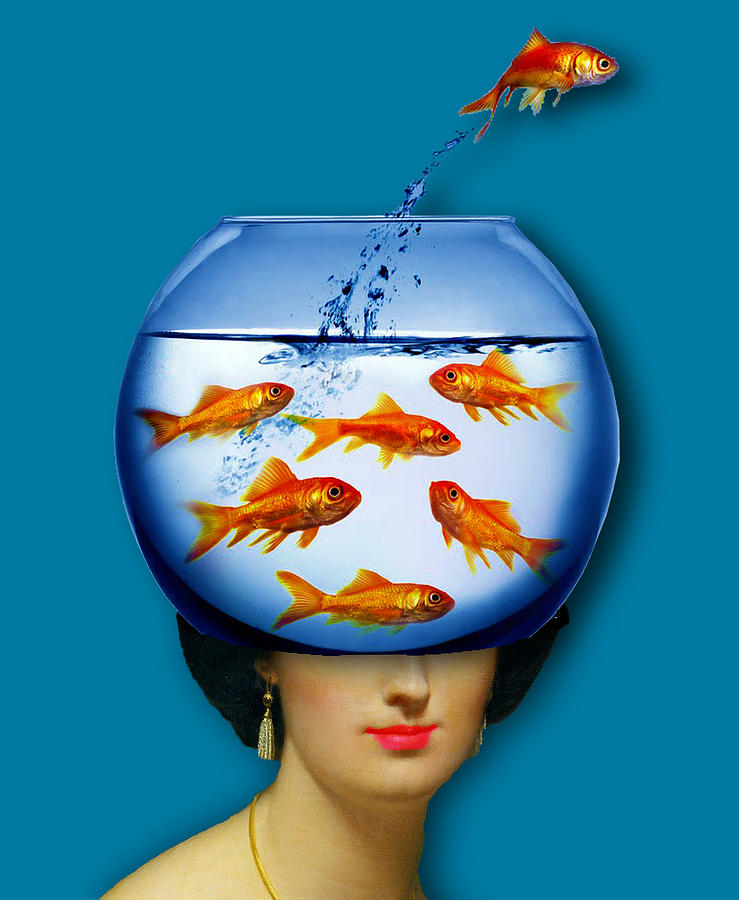In this surreal and detailed artistic portrait, the background is an aquamarine blue, enhancing the dreamlike quality of the image. The lower part of a woman's face, with pale skin and bright pink lipstick, is visible. She appears to be from a vintage, possibly Victorian era, characterized by her simple gold necklace and gold earrings with tassels. Covering her eyes, forehead, and the top of her head is a fishbowl, superimposed with a reflective and slightly glowing blue hue. Inside the fishbowl are six goldfish, some swimming contentedly while one dramatically leaps out, leaving a visible water trail as it soars towards the right. The woman has very short brunette hair, and only her right shoulder is visible, making the focus on her mysterious and otherworldly presentation.